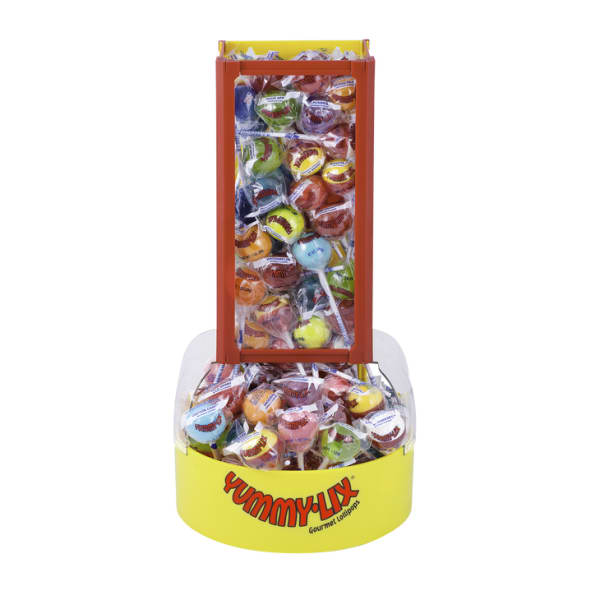This photograph features an intriguing, tower-like plastic dispenser packed with approximately 40 colorful Yummy Licks Gourmet Lollipops. The dispenser's design is divided into two main sections: a top rectangular box and a bottom square base, both transparent, revealing the multitude of lollipops inside. The top section of the box is red, while the bottom part is yellow. The lollipops come in a vibrant array of colors, including blue, yellow, red, gold, white, green, light blue, purple, pink, and orange, arranged in several rows. Prominently displayed on the dispenser is the brand name, "Yummy Licks Gourmet Lollipops," with 'Yummy Licks' in bold red letters against a yellow background, and 'Gourmet Lollipops' in smaller black font. The photo is set against a plain white background, suggesting it might be part of an advertisement.